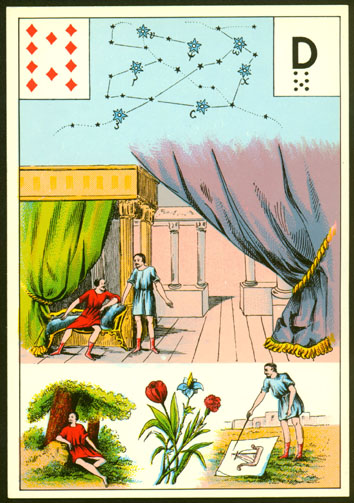The image is an intricate compilation of several distinct elements, reminiscent of a series of detailed paintings. At the top left, there is an arrangement of 10 red diamonds, configured in a pattern resembling the "10 of Diamonds" playing card, with four diamonds positioned in the corners, two in the center, and the remaining four flanking the two central diamonds. Adjacent to this, in the top right, there is a depiction of the letter "D" with seven smaller stars below it, arranged in a manner that forms an 'X' shape, giving the appearance of a constellation. This section also includes numerous smaller stars and dots connected by lines, adding to the celestial motif.

Beneath these elements, the scene shifts dramatically. Here, one can observe what appears to be a classical setting with a man seated in a cart conversing with another man who is standing beside him. This segment is framed by marble pillars and draped with elegant curtains, evoking a sense of ancient architecture and historical ambiance.

The lower portion of the compilation is divided into three distinct images. On the left, a person is portrayed sitting amidst a tree canopy, offering a serene, nature-centric scene. The central bottom image showcases three meticulously drawn flowers. Meanwhile, the bottom right scene displays a figure standing and drawing a picture, with a backdrop of intricately depicted buildings, suggesting an environment rooted in historical or ancient contexts. Each component of the image contributes to an overall sense of antiquity and classical beauty.